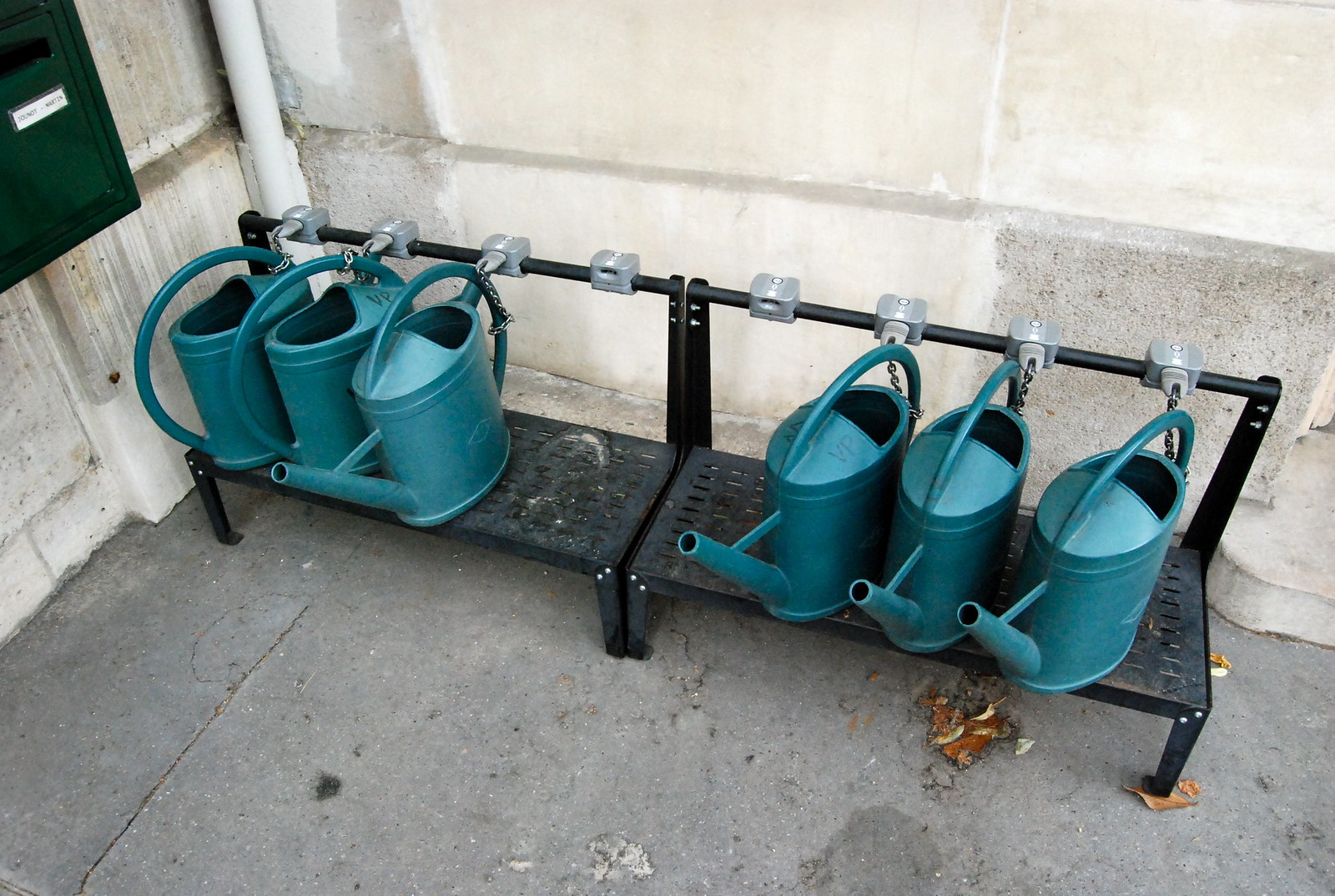The image depicts an outdoor corner where the white, somewhat dirty and porous concrete walls of a building meet. The ground is covered in grey concrete, which shows signs of aging with cracks, dark spots, and scattered dry leaves. Two black metal rails, appearing like benches with narrow slots, are positioned low to the ground against the walls. Both rails hold multiple turquoise plastic watering cans, each secured in place by a chain-lock mechanism to prevent them from being blown away or removed easily. Each rail has three watering cans, with one slot on each rail empty, indicating that two cans are in use. A white pipe runs vertically in the upper left section of the image, alongside a black box with a white rectangle on it, adding to the utilitarian feel of the scene.